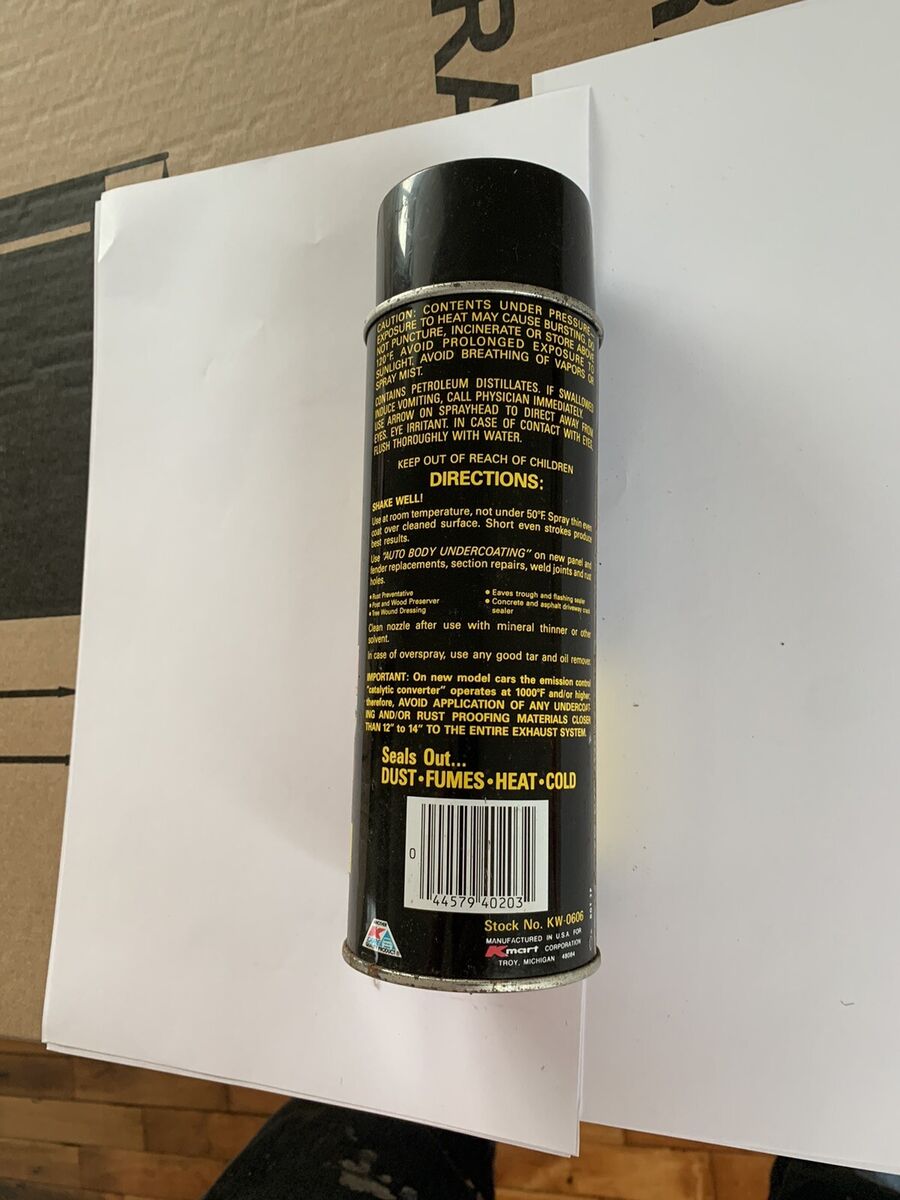The image depicts a black spray can with a silver top and bottom, and a black cap, resting horizontally on two pieces of printer paper atop a large corrugated cardboard box. The can has a portion of rust at the bottom and a barcode towards the lower section. The visible side of the can features yellow text including directions and safety warnings, stating "contents under pressure" and "exposure to heat may cause bursting." The text also highlights the can's function, mentioning that it "seals out dust, fumes, heat, and cold," indicating it is likely a type of sealant spray. The photograph is taken from an aerial perspective in portrait format, capturing the intricate details and the context of the can amidst the described setting.